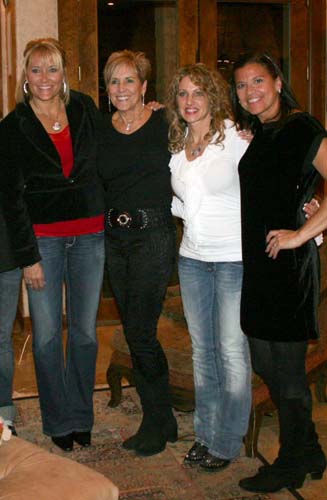Four women stand closely together in a line, each with their hands on the shoulders or sides of the woman next to them, displaying a sense of camaraderie. They are being photographed, looking slightly towards the left, with the exception of the fourth woman who gazes directly at the viewer. From left to right, their heights vary slightly, with the tallest on the far left and the shortest third in line.

The first woman on the left, with blonde hair and a fringe, wears a black jacket over a red blouse, accessorized with a silver necklace featuring a medallion and loop earrings. She pairs her outfit with blue denim jeans and black high heels. The second woman has a bob cut and sports a full black outfit consisting of a black top and black denim jeans, cinched with a black leather belt with a silver buckle. She accessorizes with long, dangly earrings and a silver necklace, completing her look with black boots.

Next is the third woman, a curly-haired brunette adorned with red lipstick. She wears a frilly white blouse, a goldish-colored necklace, and faded blue jeans, along with black shoes. The fourth and last woman, with long, straight black hair, wears a sleek black short-sleeve dress that reaches mid-thigh, complemented by black stockings, black boots, and small earrings.

The women stand on a floor covered with an oriental rug featuring red, blue, and green patterns, hinting at a setting that could be a restaurant or hotel. Behind them hangs a dark-colored curtain, perhaps burgundy or brown, blurred in the photograph's dim lighting. They all smile warmly, suggesting a shared moment of friendship or celebration.